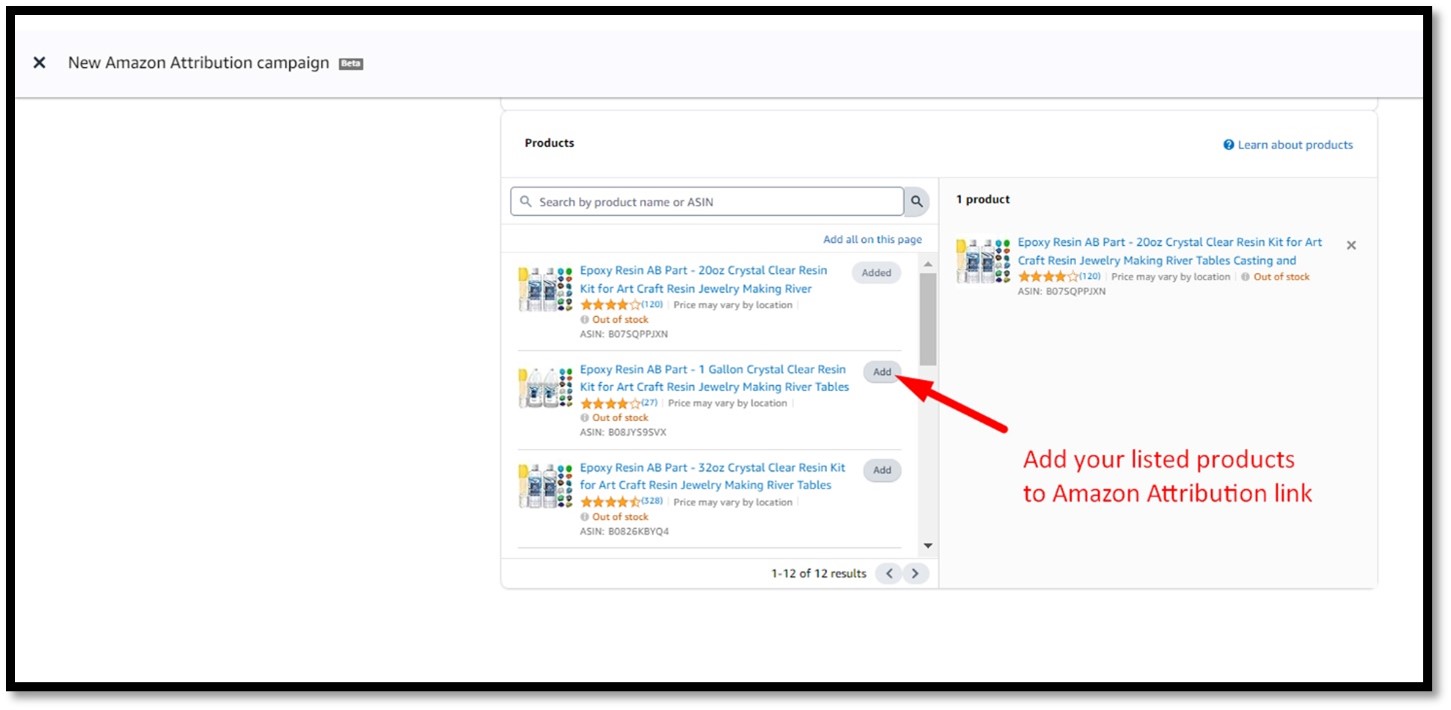This image appears to be a screenshot from a website showcasing a product listing interface, potentially from Amazon's Attribution campaign tool. The image is bordered by a black edge with a slight grey shadow underneath, giving it a framed effect. 

At the top left corner, there is a small "X" button, suggesting an option to close the current view. Next to it, bold text reads "New Amazon Attribution Campaign," accompanied by a small rectangle to its right containing unreadable white text. Below this header, a grey horizontal line spans the image, slightly off-center, dividing different sections.

On the left side, there is a blank rectangle beneath the horizontal line, possibly a placeholder for additional content. The center of the image features a table layout. At the top of the table, the word "Products" is prominently displayed in black, while a blue text link reading "Learn About Products" is positioned to the right.

The table lists several products, starting with "Epoxy Resin, 20cc Crystal Clear Resin Mix for Craft, Jewelry Making," which is rated with four stars. The product below is a similar item described as "Gallon Crystal Clear Epoxy Resin Kit." Another product at the bottom is a kit for aircraft construction, with an image including bottles of resin in various colors on the left and a yellow-handled applicator tube on the right.

Below these product listings, the image indicates "1-12 of 12 results," suggesting the current page view of the product list. To the right of this text, there is a product similar to the top-listed epoxy resin, described as "Epoxy Resin, 48 Port, 20 oz Crystal Clear Resin, 10cc for Art, Craft Resin, Jewelry Making, River Tables, Clothing."

At the top right corner of the image, a "Learn About Products" link is also present. Additionally, red overlay text on the website instructs users with "Add your listed products to the Amazon Attribution link," accompanied by a red arrow pointing to the second product in the row of three on the left side, directing attention towards an "Add" button on the right.

Overall, this detailed screenshot provides a comprehensive view of an Amazon Attribution campaign tool, showcasing various resin products, with functional links and instructional overlays to guide users through the interface.